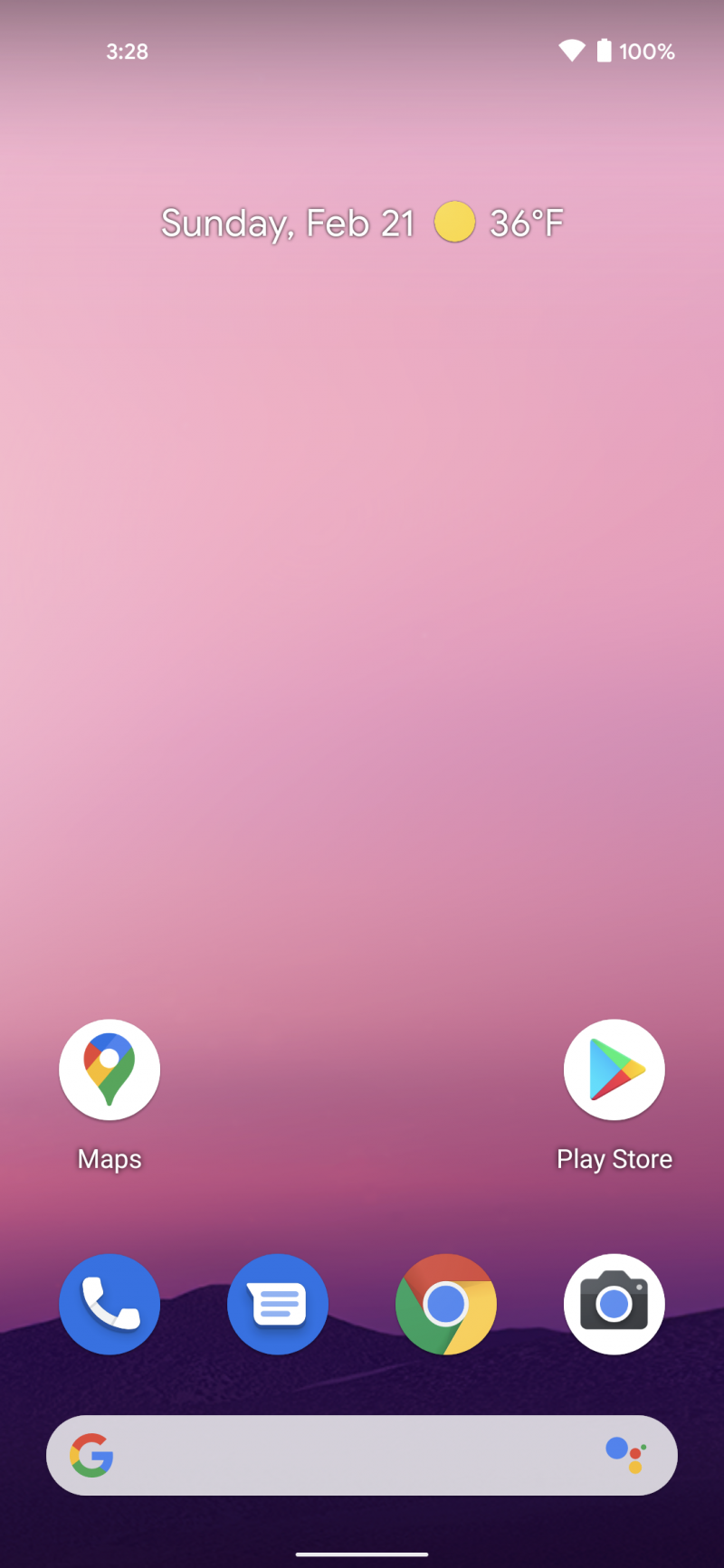The screenshot displays a typical smartphone home screen with various status indicators and app icons. In the top left corner, the time is shown as 3:28, while the top right corner shows a full battery at 100% and a fully connected Wi-Fi signal. The background is a gradient of pink, transitioning to dark purplish hues at the bottom, resembling mountains.

Below the time, there is a date display showing "Sunday, February 21st" along with a sun icon and the temperature reading "36°F". Moving further down, several app icons are lined up. From left to right, they include:

- A map icon with a varied color pinpoint (green, blue, red, yellow)
- The Play Store icon featuring a right-pointing arrow in cyan, blue, pink, red, and yellow
- A phone call icon
- A text message icon
- The Google Chrome browser icon with its characteristic yellow, green, red, and blue sections
- A camera icon

At the very bottom of the screen is a search bar with the Google logo, marked by the colorful 'G' (blue, green, yellow, red) and additional blue, red, yellow, and tiny green circles. In total, there are six app icons displayed on the screen.